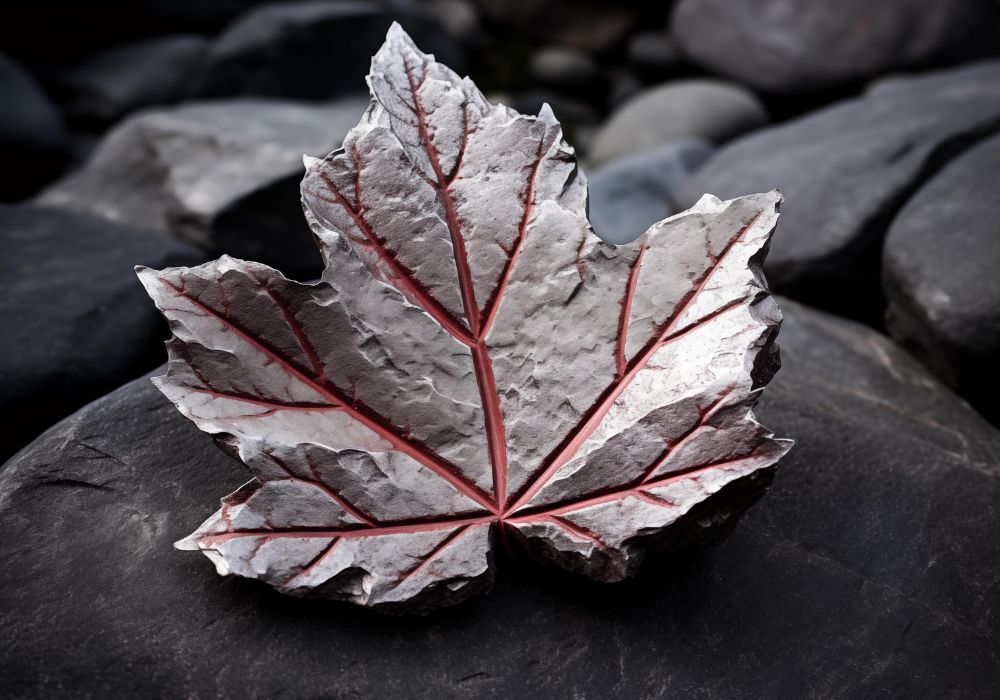The image depicts a close-up scene dominated by a collection of large, dark granite rocks that form a strikingly deep black and gray background. Centered prominently in the foreground, perched atop one of these rocks, is a meticulously carved stone leaf. This leaf, rendered in a light ash gray color, features intricate red veins etched deeply into its surface, mimicking the natural vein structure of a typical tree leaf. The leaf, which lacks a stem, appears almost metallic or fossilized, providing a stark yet harmonious contrast to the darker hues of the surrounding rocks. The red veins add a vivid highlight, drawing the viewer's attention and emphasizing the leaf's detailed craftsmanship against the textured, shadowy backdrop.